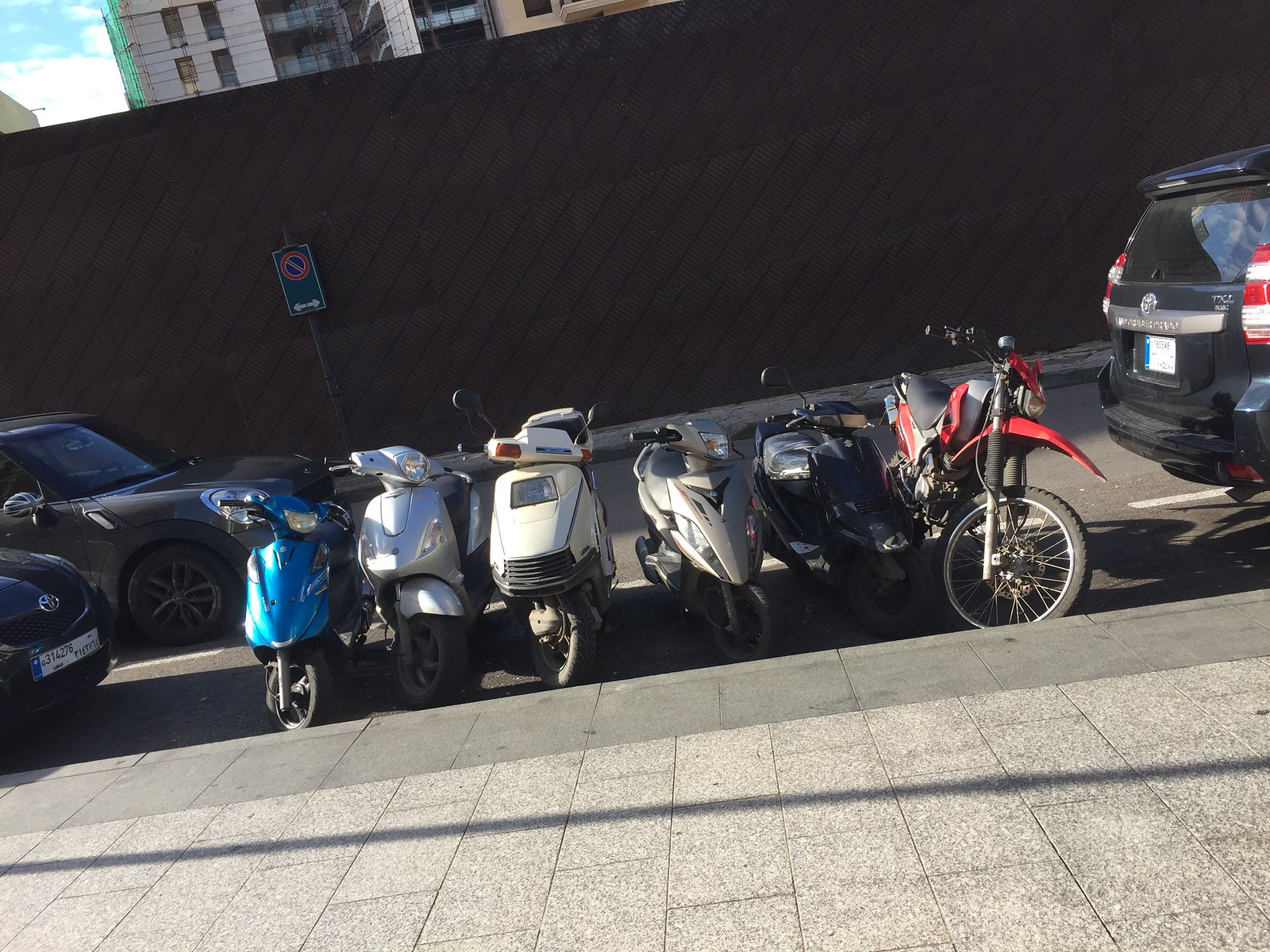This outdoor color photograph, taken on a sunny day with a blue sky dotted by sporadic white clouds, captures a lively street scene. The background features a large white building, possibly an apartment complex or business, with numerous windows. In front of this building stands a sizeable reddish-brown wall with diagonal boards, resembling a privacy or sound barrier. 

Dominating the scene is a parking area along the sidewalk, constructed with textured concrete or granite slabs arranged in a brick pattern. Casting shadows, likely from street lights or power lines, stretch across the frame. 

Prominently, there’s a blue metal street sign mounted on a brown pole near the wall. The sign displays a red slash through a circle, indicating "no parking," with a white arrow pointing in both directions. 

Lined up along the curb are six motorcycles, parked front-facing, in designated parking spots. They range in colors and styles: an electric blue scooter/moped, a white motorcycle, a tan bike with a wide front grille, a sporty silver bike, another sporty black one, and a red and black dirt bike with upright handles. 

Adjacent to these motorcycles, a Toyota SUV, likely a Highlander, is parked, revealing only its rear with the logo visible. Two other cars are parked nearby, positioned in the same direction as the SUV, while the motorcycles are aligned differently for clear front views. The photograph captures the intricate details of urban street life on a sunny day, marked by shadows and reflections on the street surface.